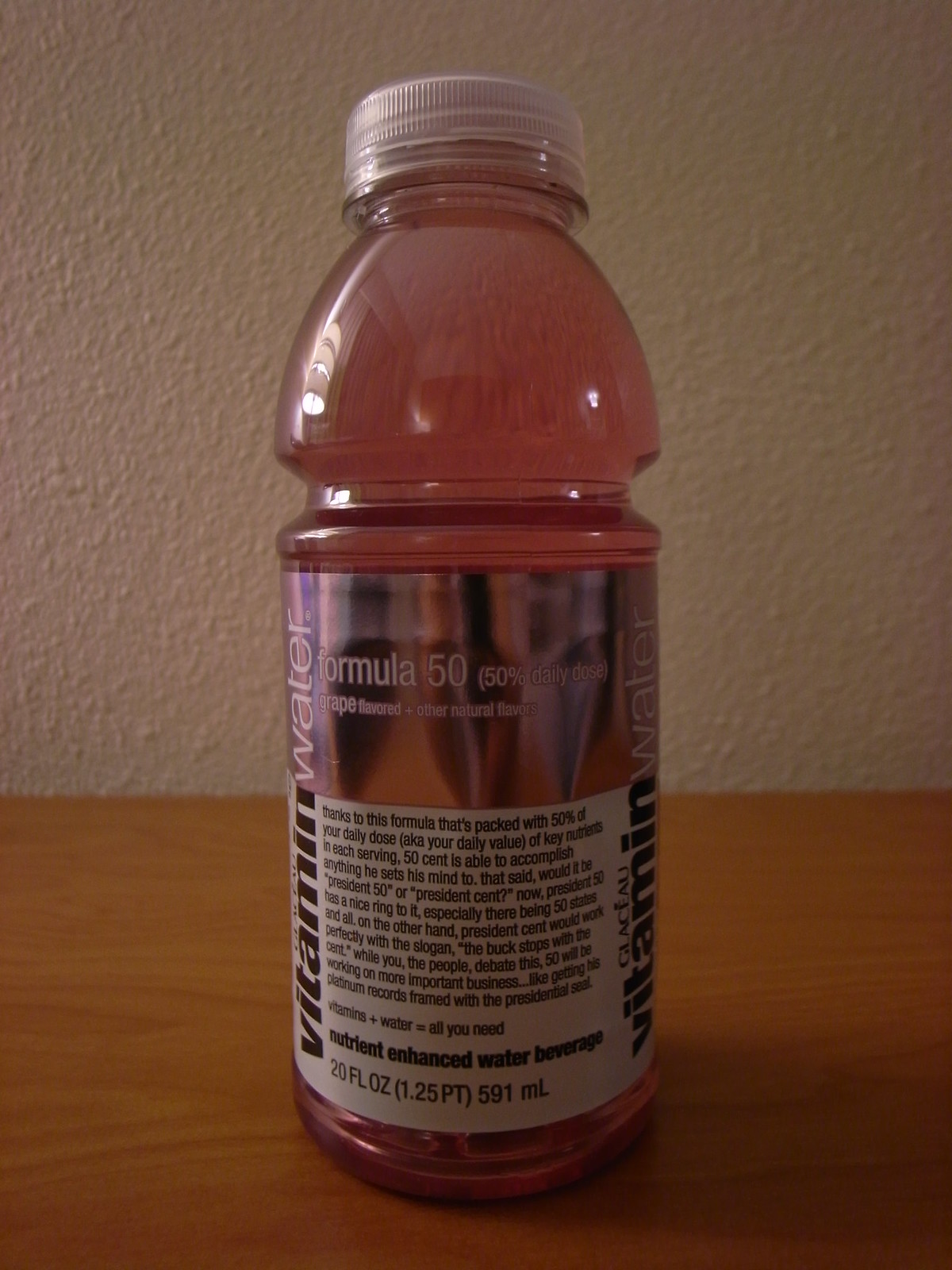A vibrant purply-pink bottle of Vitamin Water, containing 20 fluid ounces (591 milliliters), stands out with its eye-catching design. The bottle’s label, with a sleek metallic finish, prominently highlights its contents, boasting that each serving provides 50% of the daily value of key ingredients. The playful blurb on the label notes that with this fortified formula, even the rapper 50 Cent is empowered to achieve his goals, pondering humorously whether he should be called President 50 or President Cent. This detailed packaging merges functionality with a touch of whimsy, making it both informative and entertaining.